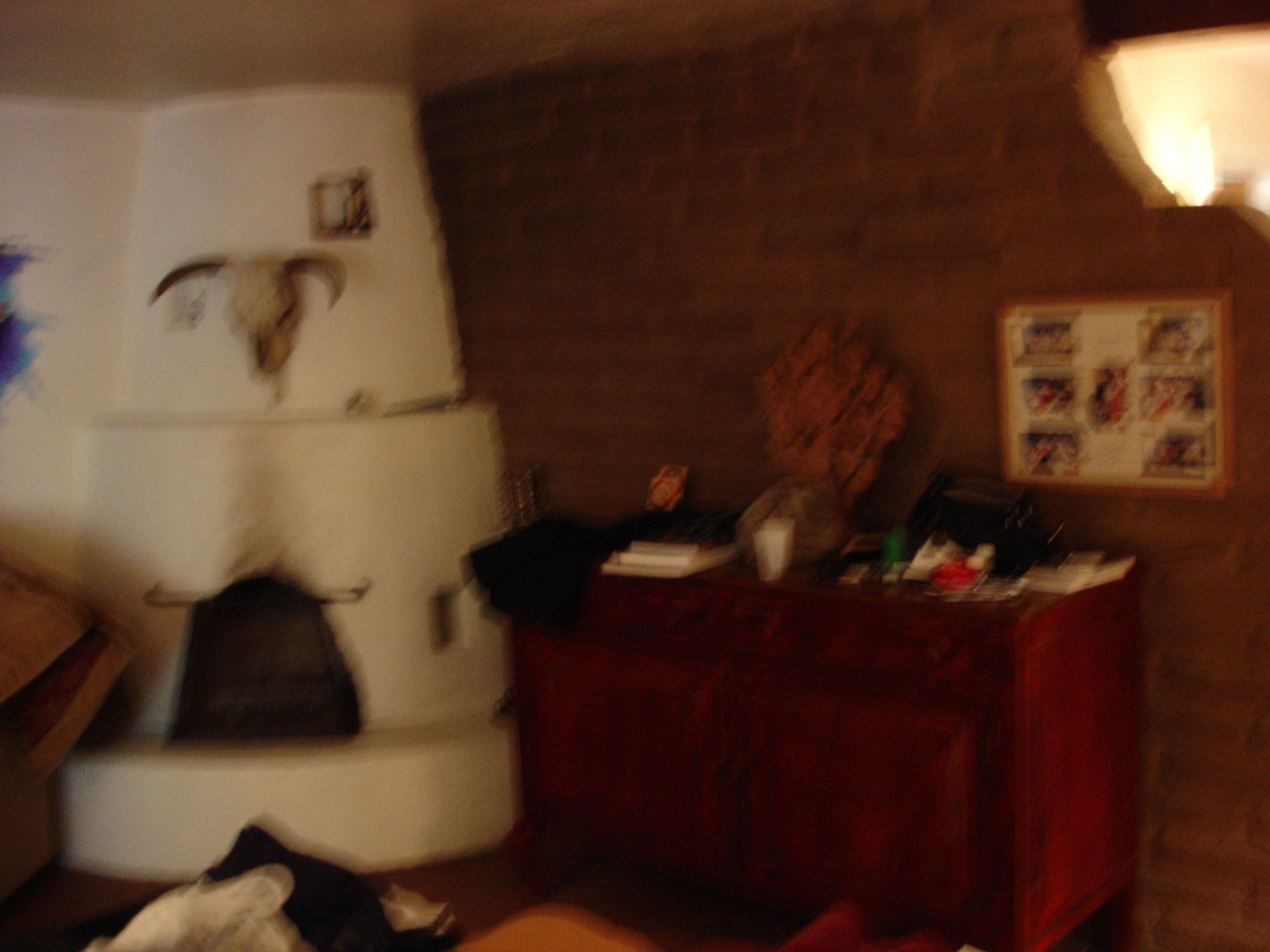The image depicts a dimly lit living room, shrouded in shadows, and characterized by dark browns, whites, and hints of reddish-brown and orange hues. Dominating the center of the scene is an adobe-style fireplace, adorned with an imposing cattle skull. To the left of the fireplace, a framed picture hangs on a brick wall, its details indistinct due to the blur. Along the right side of the room stands a brown cabinet, topped with an array of items including flowers, books, and other indiscernible objects. The cozy yet somewhat mysterious ambiance is accentuated by the room's rustic decor elements.